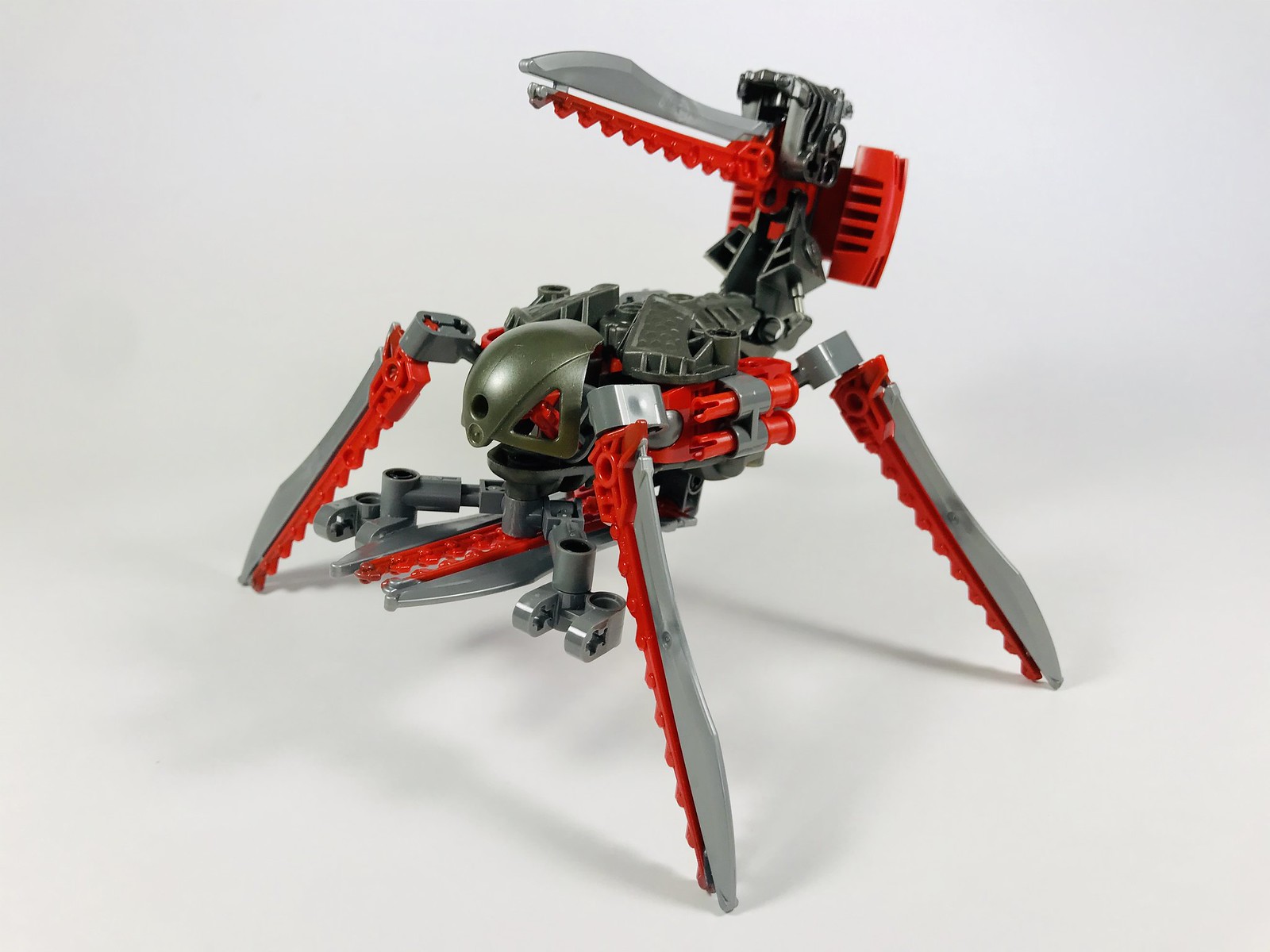This detailed photographic image depicts an intricately constructed Lego creature set in an indoor environment with a grey shadowed background. The creature boasts four grey and red legs designed with zigzag patterns and tapered ends, providing sturdy support to its grey engine-like body, accentuated by red side pistons. Beneath the main body lies a cylindrical element flanked by two additional legs, alongside a jaw-like structure featuring a grey exterior and a red interior, reminiscent of a menacing mouth. The top of the creature showcases a unique key or saw-like extension; this part includes a horizontal red saw-tooth design and a vertical black piston that stands erect. Additionally, there seems to be a long beak-like neck pointing towards the upper left corner of the image, suggesting a creature-like appearance. The ensemble is completed by a helmet-shaped piece at the front, adding an intricate detail that contributes to the overall mechanical and somewhat organic aesthetic of the Lego creation.